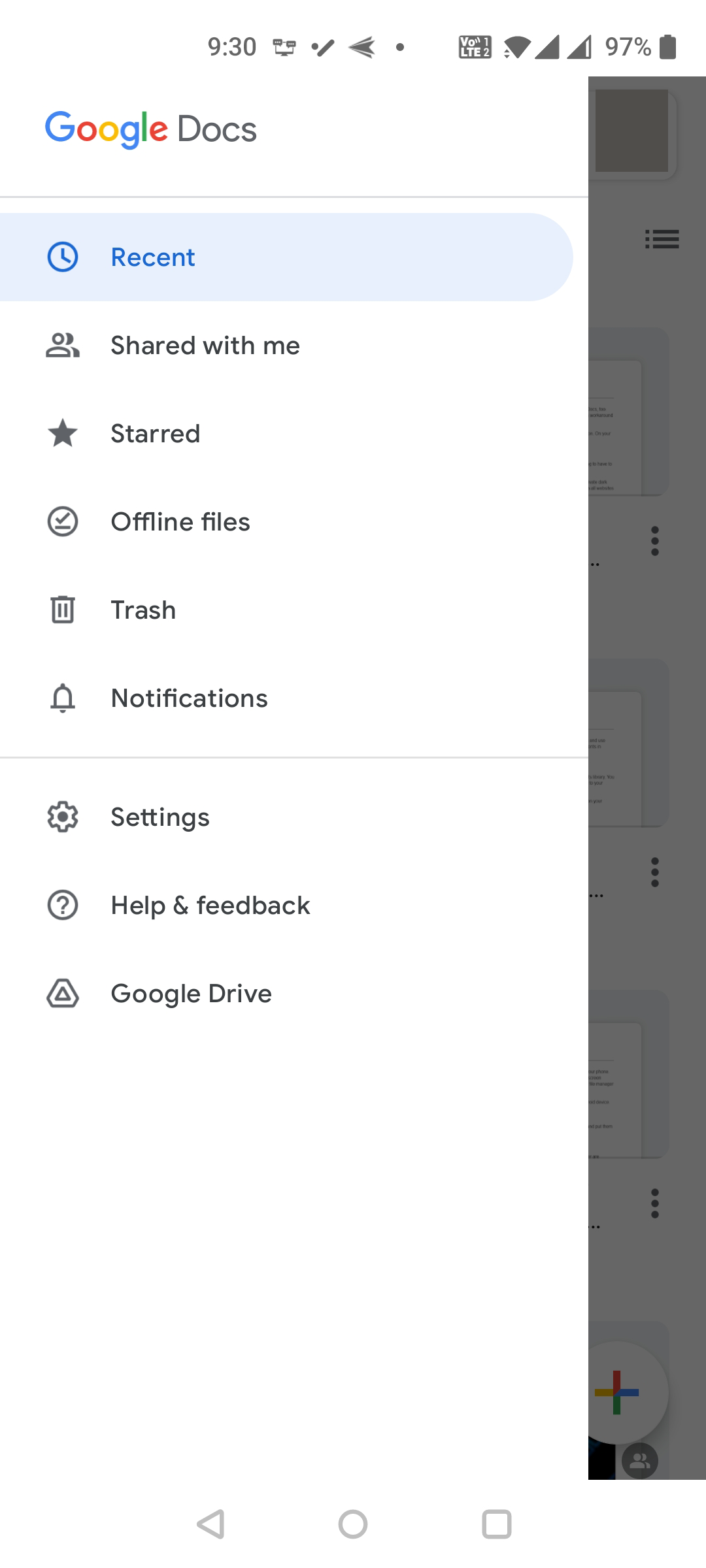This screenshot captures the navigation menu from the Google Docs mobile app, offering a comprehensive view of its functionalities. The menu options displayed include:

- **Recent**: Access recently viewed documents.
- **Shared with Me**: View documents shared by other users.
- **Starred**: Access documents you've marked as important.
- **Offline Files**: View documents available without an internet connection.
- **Trash**: Access deleted documents.
- **Notifications**: Configure your notification settings.
- **Settings**: Customize app preferences.
- **Help and Feedback**: Seek assistance or provide feedback on the app.
- **Google Drive**: Directly navigate to Google Drive.

The bottom section exhibits standard Android navigation icons for **Back**, **Home**, and **App Switcher**. The device's status bar shows a battery level of 97% and the time as 9:30. In the background, vague outlines of document thumbnails are visible, indicating the presence of various documents, though specific content is indiscernible.